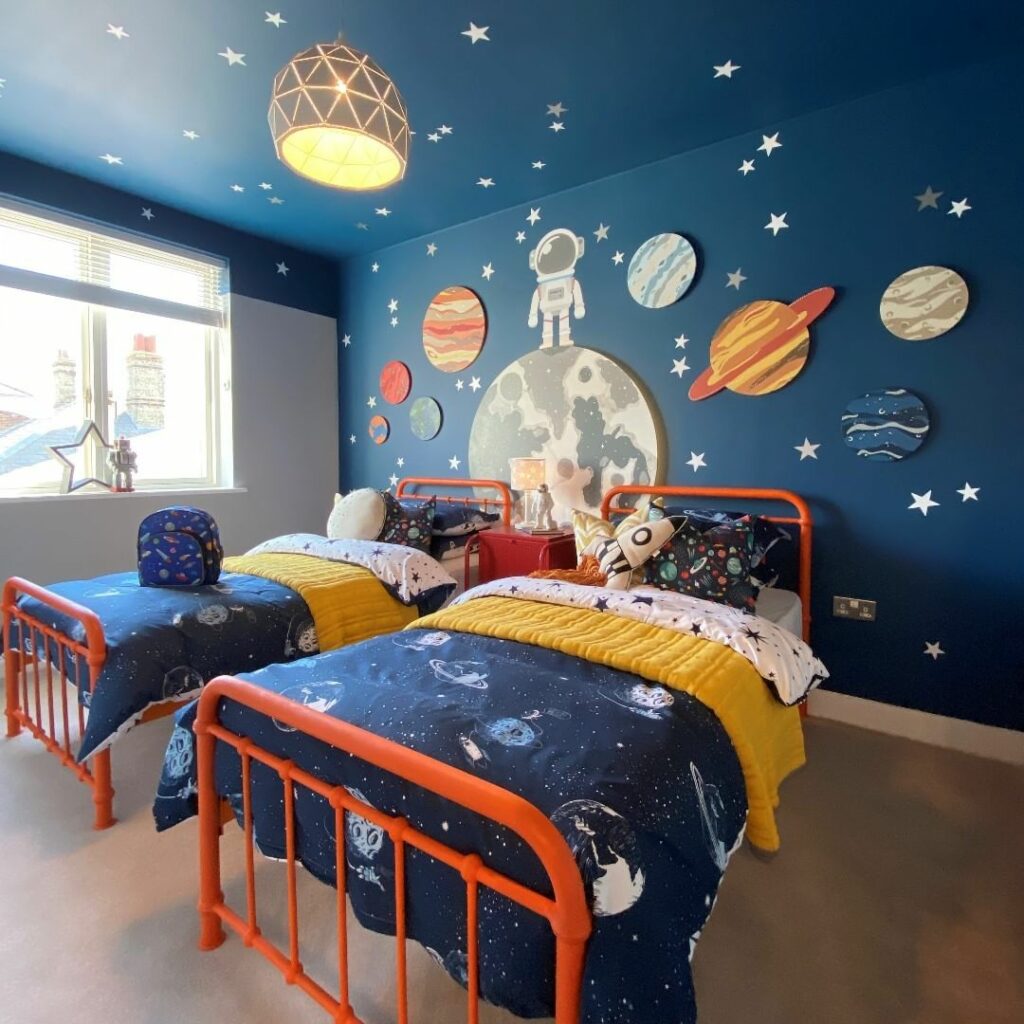The image shows a cozy children's bedroom designed for possibly two young siblings, with an appealing space theme that features prominently throughout the room. Centrally positioned are two beds with matching blue bedspreads adorned with galaxy-themed patterns. Each bed also includes a yellow comforter and a long white pillow. The beds are supported by identical orange frames, which appear to be made of a painted PVC pipe.

The right wall stands out with a vivid blue backdrop, artistically decorated with colorful cutouts of planets, stars, and a cartoonish astronaut standing on what appears to be the moon, evoking a playful outer space environment. This celestial motif extends across the ceiling, enhancing the room's immersive experience. To the left of the beds is a window, and above, a yellow light fixture illuminates the room, adding to the warm and inviting atmosphere. The overall aesthetic is that of a well-loved space-themed haven for two young children, potentially fostering their imagination and love for the cosmos.